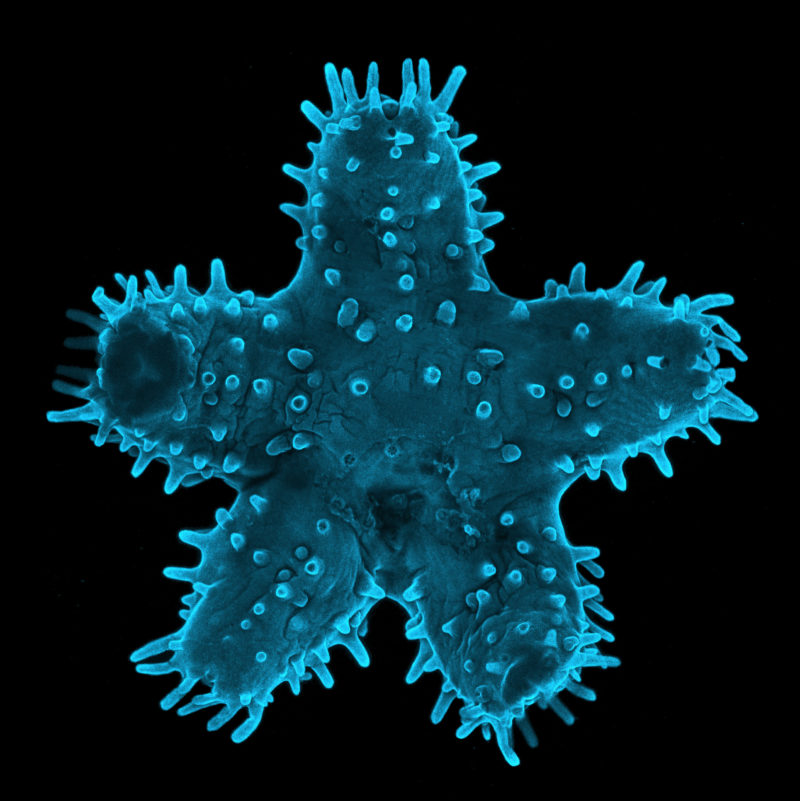The image showcases a striking illustration of what appears to be a sea creature, resembling a starfish, set against a deep black background. The creature exhibits a vivid blue coloration with nuanced shades ranging from light blue at its edges to darker blue across its main body. Characterized by a five-legged star shape with one limb positioned at the top and two at the bottom, the surface of the creature is adorned with numerous small tubules or spiny projections. This detailed depiction gives the impression of either a microscopic view of a real organism—potentially a parasite, amoeba, or starfish—or a digitally crafted image, with its precise, vivid colors sharply contrasting against the dark backdrop for emphasis.